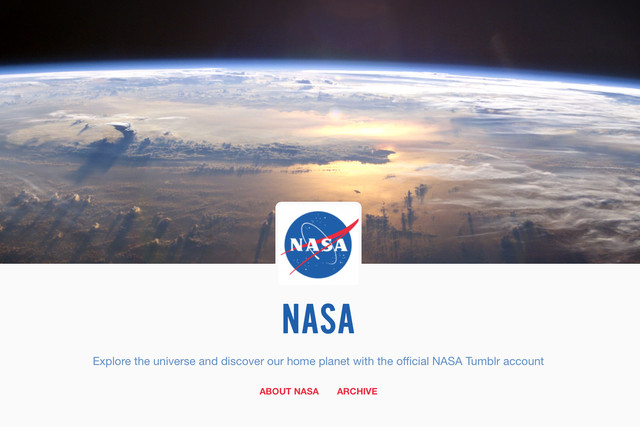This cropped screenshot showcases the header from NASA's official Tumblr account. Dominating the header is a high-definition image of Earth, where the planet's curvature is clearly visible against the stark blackness of space. The bottom center of the image features a large, semi-transparent square that extends out of the frame. Within this square is the prominent NASA logo, with the word "NASA" displayed in bold, blue capital letters beneath it. Directly below the logo, in smaller blue font, is the phrase: "Explore the universe and discover our home planet with the official NASA Tumblr account." Beneath this tagline, centered in red font, the links "About NASA" and "Archive" are positioned on the lower left and right, respectively. The rest of the Tumblr page is cropped out, focusing solely on the striking visual and succinct introductory text within the header.